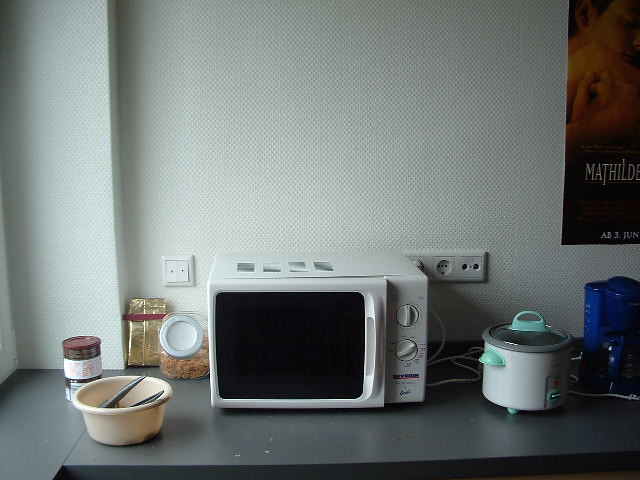The image depicts a modest European kitchen setup, possibly within a small apartment or office space, featuring mainly gray and white tones. Central to the scene is a white, older-style microwave with two knobs and a black glass door, positioned on a dark gray or black countertop. To the microwave's right sits a white rice cooker or slow cooker with lime green handles and buttons. To its left, there's a collection of containers, including jars possibly filled with pasta and rice, and a small brown bowl containing cooking utensils. The backdrop is a textured white wall adorned with a partially visible poster that reads "Mathilde," likely indicating a movie poster. European-style outlets and switches are also visible on the wall. Light appears to enter from the left side of the image, suggesting the presence of a window.